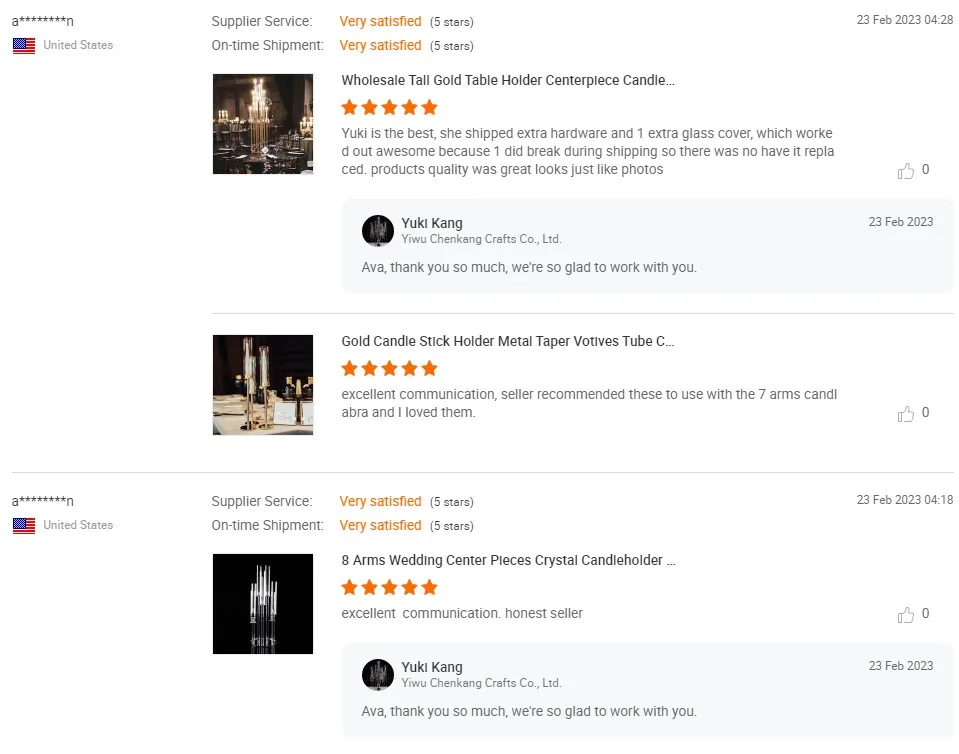In the image, we see a customer review page showcasing multiple user reviews. One review, posted by Eva on February 23rd, 2023 at 4:28 PM, rates the product with 5 stars and praises Yuki for exceptional service. Eva mentions that Yuki included extra hardware and an additional glass cover, which proved to be beneficial since one glass cover broke during shipping. Eva appreciates the product's quality and attests that it matches the photos provided.

Yuki Kang from "Yui Cheng Kang Craft Co. Ltd" has responded to Eva's review, expressing gratitude and joy for the opportunity to work with her.

The second review, also posted on February 23rd, 2023, rates a gold candlestick holder with a metal tip and voltage tube with 5 stars. The review commends the seller's excellent communication and mentions that Yuki recommended using it with a 7-amp candelabra, which the reviewer loves.

A third review below echoes similar sentiments about Yuki's excellent communication and honesty, accompanied by another 5-star rating. Yuki responds once again, thanking Eva and expressing her pleasure in working with her.